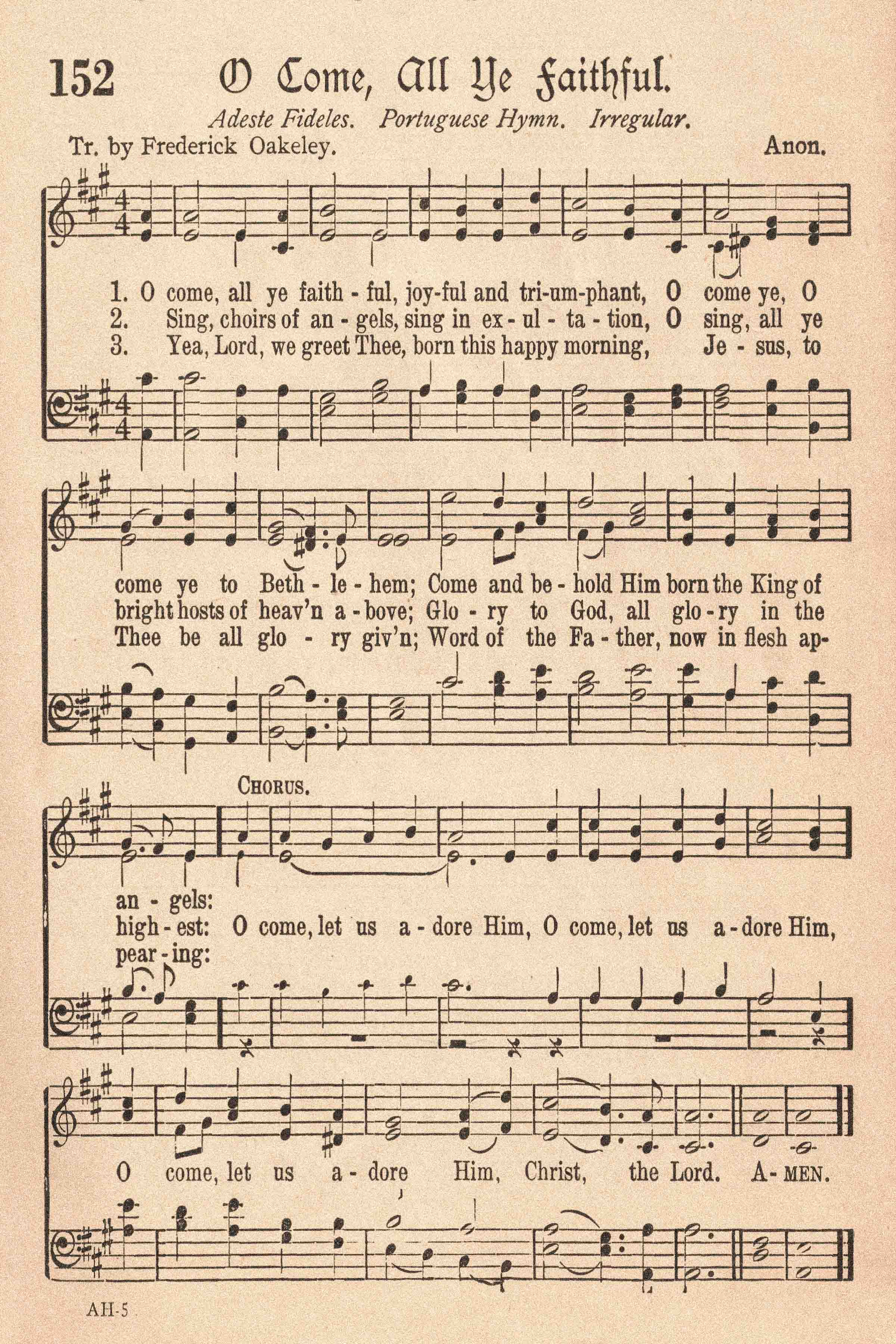The image depicts a scanned sheet of music on a beige or tan colored piece of paper titled "152 O Come All Ye Faithful." The title is followed by the note "Adeste Fidelis" indicating the Portuguese hymn, with an irregular meter, and translated by Frederick Oakley and Anon. The sheet features multiple lines of musical notes and printed black lyrics for the song. The lyrics start with "O come all ye faithful, joyful and triumphant. O come ye, O come ye to Bethlehem. Come and behold him born the King of Angels. O come let us adore him, Jesus Christ the Lord. Amen." This is followed by "Sing, choirs of angels, sing in exultation. O sing, all ye bright hosts of heaven above. Glory to God, all glory in the highest. O come, let us adore him. O come, let us adore him." The final verse reads, "Yea, Lord, we greet thee, born this happy morning." The overall presentation of the sheet includes many lines of music and printed lyrics, providing detailed instructions for both playing and singing the song.